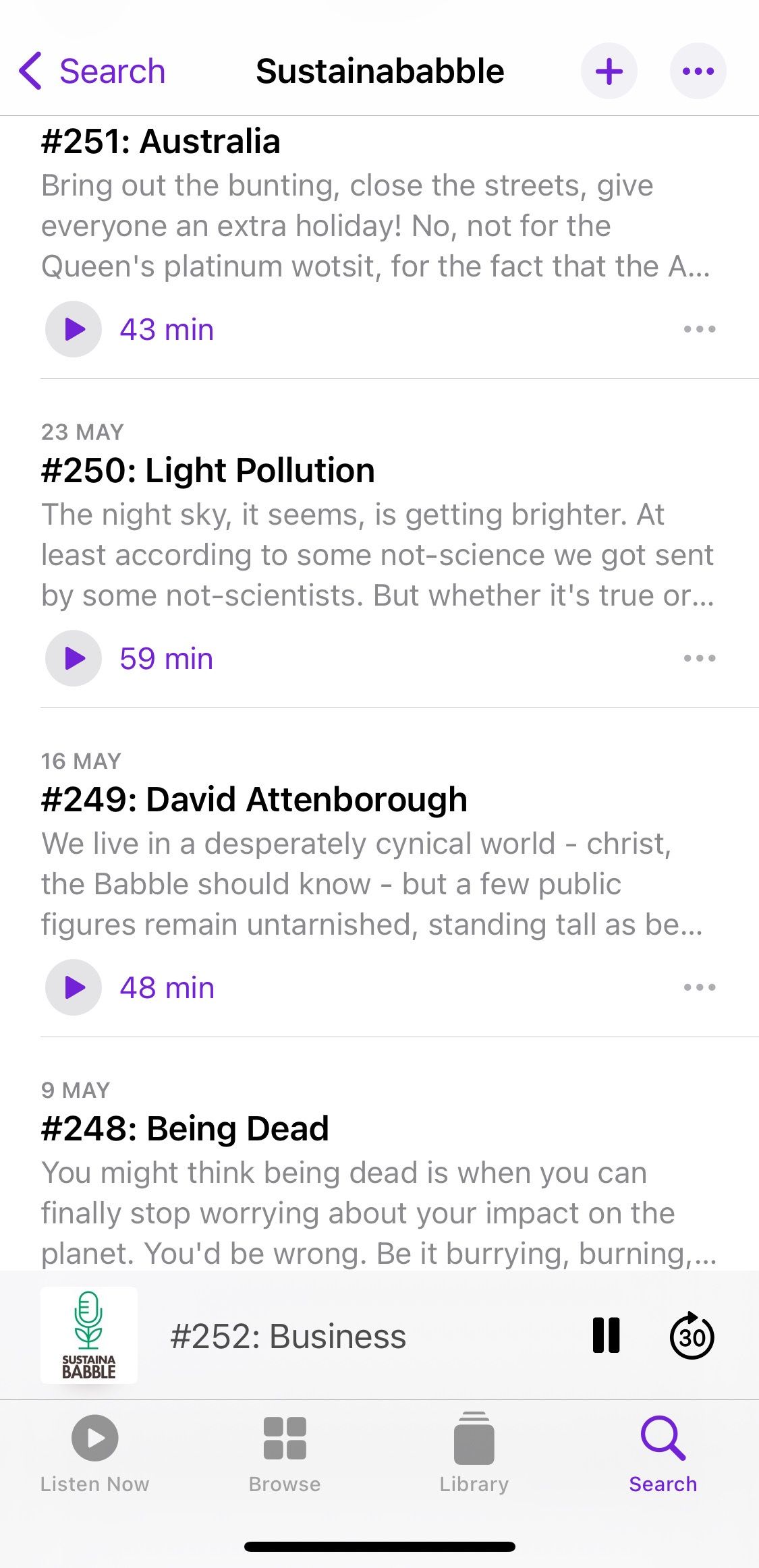Here's a cleaned-up and detailed caption for the image:

---

The image displays a search results page from an audio streaming or podcast application. At the bottom of the screen, there is a navigation bar with four options: "Listen Now," "Browse," "Library," and "Search." The "Search" option is highlighted in purple, while the others are in grey. 

At the top of the page, there is a search bar accompanied by a left-pointing arrow. Below the search bar, the phrase "Sustain A Babble" is written in bold black letters, followed by a plus sign and a menu icon represented by three vertical dots.

The first search result is labeled as Episode 251, titled "Australia: Bring out the bunting, close the streets, give everyone an extra holiday. No, not for the Queen’s Platinum Jubilee, but for the fact that the A..." There is a play button indicating the episode length of 43 minutes, and the release date is noted as May 23.

Further down, there is another entry, Episode 250, titled "Light Pollution: The night sky is getting brighter, at least according to some non-scientists..." This episode also has a play button with a duration of 59 minutes and was released on May 16.

Another listed episode is Episode 249, featuring David Attenborough, with the title "We live in a desperately cynical world. Christ, the babble should know, but a few public figures remain untarnished, standing tall..." The play button indicates a duration of 48 minutes, and it was released on May 9.

The final visible episode in the list is Episode 248, simply titled "Being Dead," with no additional details provided in the visible text.

---

This caption provides a clear and detailed description of the visual elements and content presented on the search results page.